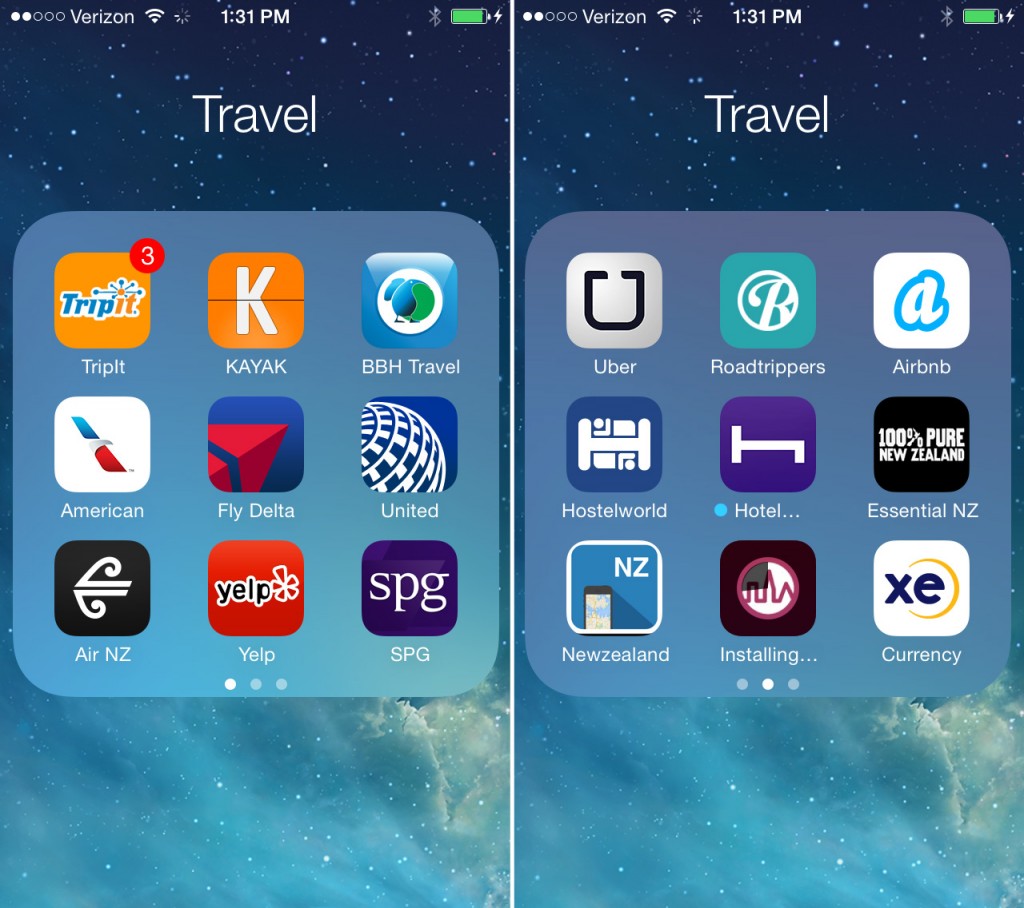The image is a comparison of two phone screenshots, each displaying their respective home screens. Both screens show the same time, 1:31 PM, alongside the Verizon network indicator and a full battery icon. The top of each screen also features a "Travel" label, suggesting these are travel-related apps.

On the left screenshot, nine icons are neatly arranged into three rows of three. The top row features "TripIt" on the top left, "Kayak" in the center, and "BB-8 Travel" on the top right. The second row includes "American Airlines" on the left, "Fly Delta" in the center, and "United Airlines" on the right. The bottom row showcases "Air NZ" on the left, "Yelp" in the center, and "SPG" on the right. Each app is represented by its respective logo.

The right screenshot also displays nine icons in a similar three-by-three grid. The top row consists of "Uber" on the left, "Roadtrippers" in the center, and "Airbnb" on the right. The second row contains "Hostelworld" on the left, "Hotel Essentials" in the center, and "NZ Travel" on the right. The bottom row has icons for "New Zealand" on the left, "Installing" in the center, and "Currency" on the right.

Each icon within the grids is represented by its respective app logo, maintaining visual consistency and aiding in quick identification for the user.